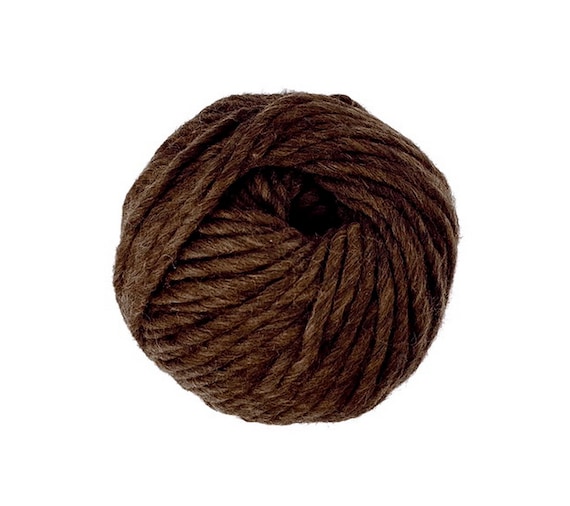This color photograph features a compact, ball of brown yarn set against a plain white background, which makes it stand out distinctly. The yarn is tightly wound, with no visible loose ends, and is slightly irregular in shape, reflecting its natural texture. Various shades of brown, cream, and darker hues can be seen throughout the ball, adding depth and interest. The strands of yarn are thin, about the thickness of shoelaces, and they weave together to form a ball-like appearance with a noticeable small divot at the top center. The texture appears gritty yet soft, emphasizing its cloth-like, fibrous quality. The simple composition focuses solely on the ball of yarn, with no other elements such as text, people, animals, buildings, or vehicles present in the image.